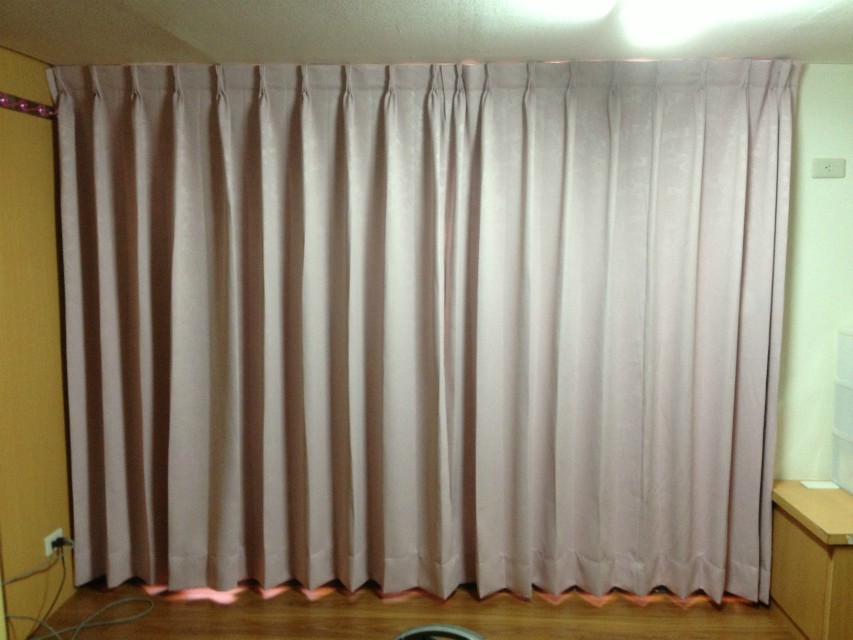The photograph predominantly features an extensive, pleated curtain in the foreground, extending from ceiling to floor. The curtain, which is likely an off-white or light gray color and made of cotton fabric, appears worn and has been hanging for a while. It spans nearly the entire width of the image, presumably covering a window or serving as a room divider. To the left, a wooden door and wall can be seen, complemented by a matching polished hardwood floor below. An outlet located at the bottom left of the image has several cords plugged in. On the right side, a wooden bench area is visible alongside a light mint green wall. The scene is illuminated by a bright light near the ceiling on the right, casting a lighter hue on that side of the room while leaving the left side slightly darker.